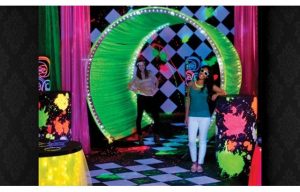The image depicts a small, low-resolution photograph featuring two young women, possibly teenagers or tweens, in an interior room with a retro neon theme. The setting resembles an arcade, laser tag venue, or funhouse, characterized by a black and white diagonal checkered floor and wall pattern. Central to the composition is a glowing neon green circular tunnel or archway, flanked by bright pink and green curtains. The girl in the foreground, positioned fully under the archway, sports sunglasses, a thick golden necklace, a teal tank top, and white pants. She has long, dark brown hair. The second girl, standing near the tunnel's entrance, also wears glasses, a pinkish-purple shirt, black pants, and has straight long hair. Scattered around the scene are black objects, possibly barrels, splattered with neon paint, and a round table covered with a yellow drop cloth in the lower left corner. The overall vibe is chaotic and colorful, consistent with a fun, playful environment.